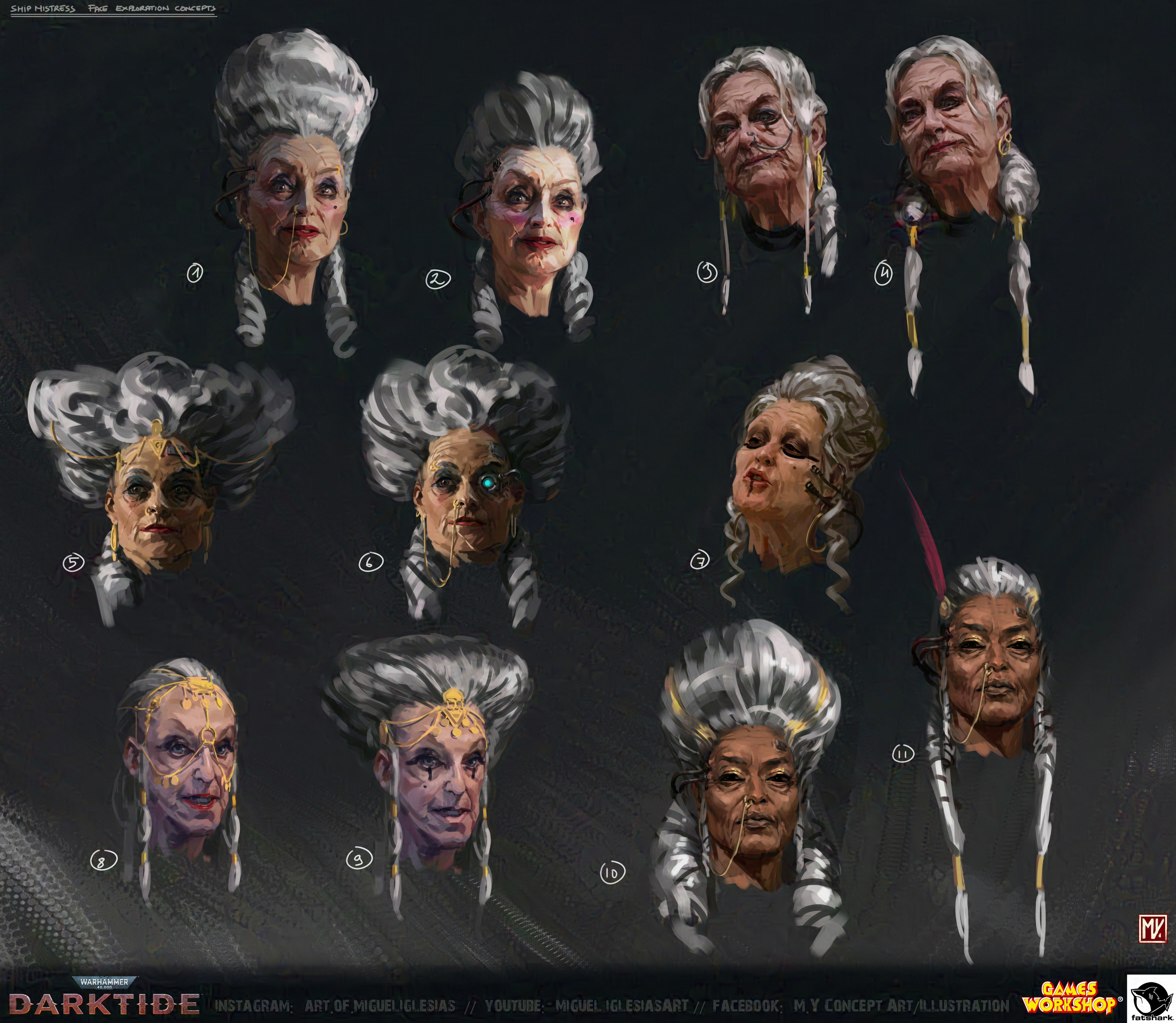The image advertises Warhammer 40k: Darktide and features 11 to 12 portraits of women's faces, all predominantly centered and scattered across the picture. Each face appears decrepit and somewhat terrifying, characterized by their gray hair styled in elaborate updos and bouffants, with some showing braided hairstyles. The women wear heavy makeup, including dark eye shadow, pink blush, and red lipstick. The skin tones vary slightly, but most faces seem to depict white women, with one noticeable black female character. The background colors are shades of gray, beige, tan, black, darker red, yellow, and pale red. At the bottom of the image, various text details credit Miguel Iglesias for the concept art, mentioning platforms like Instagram, YouTube, Facebook, and linking to 'MY Concept Art/Illustrations'. The Games Workshop logo, along with the names Gameworks and Fatshark, is visible in the lower corners, indicating the creators and publishers behind the artwork.